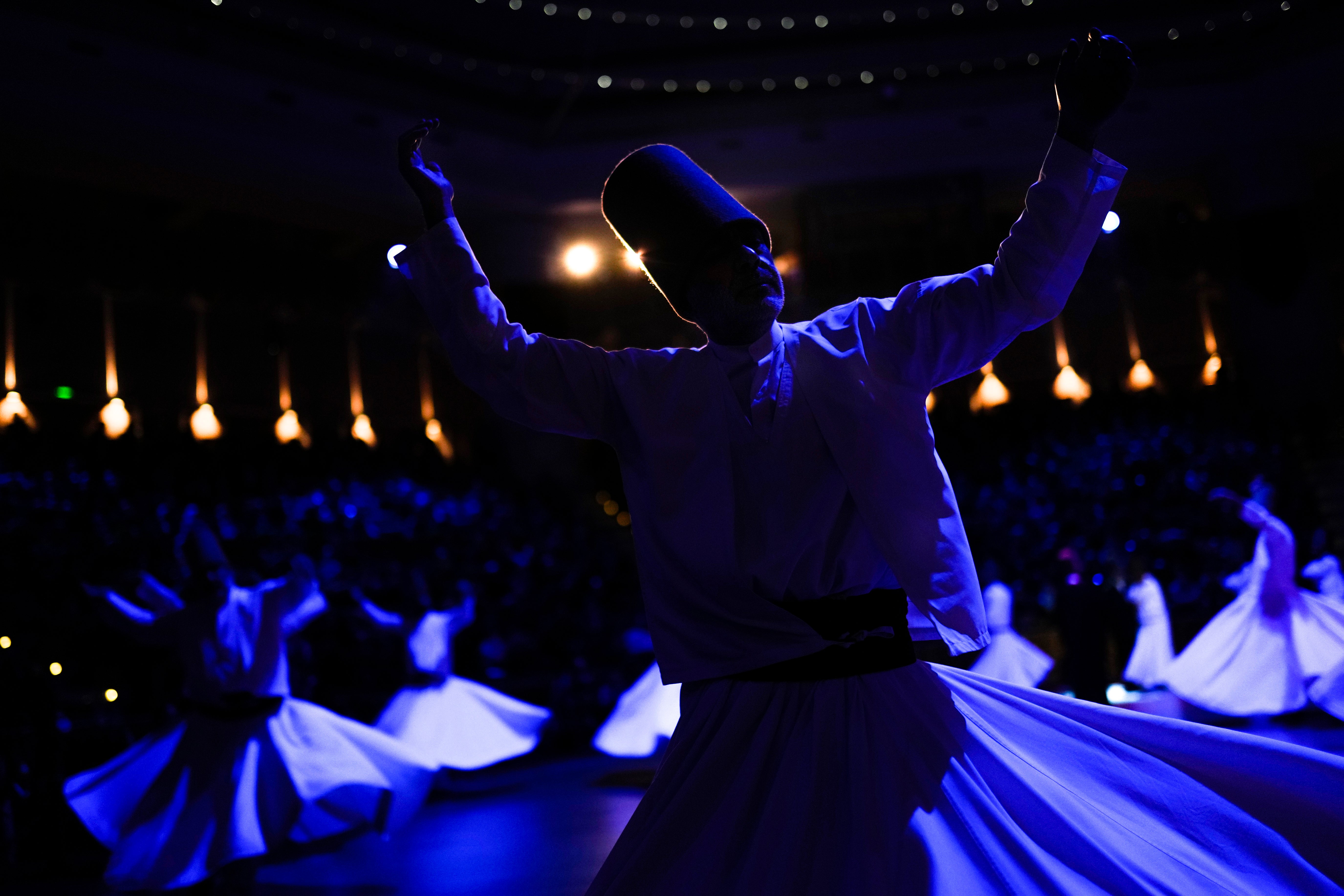The photograph captures a horizontally extended image of a dimly lit dance performance featuring Middle Eastern dancers. Dominating the foreground is a man dressed in a purple outfit, consisting of a flowy skirt, a tall cylindrical hat, and a blazer, with both arms raised as he spins gracefully. The background is hazy but illuminated with a mixture of dark blue and beige lights, creating a spotlight effect at the top center, and lines of warm orange lights flanking the sides. Fading into the darkness, other performers in similar attire can be seen arranged in circular formations, their skirts flaring out as they twirl. The audience is vaguely visible, shrouded in blue light, suggesting the grandeur of a large, multi-leveled stadium embracing the atmosphere of this mesmerizing performance.